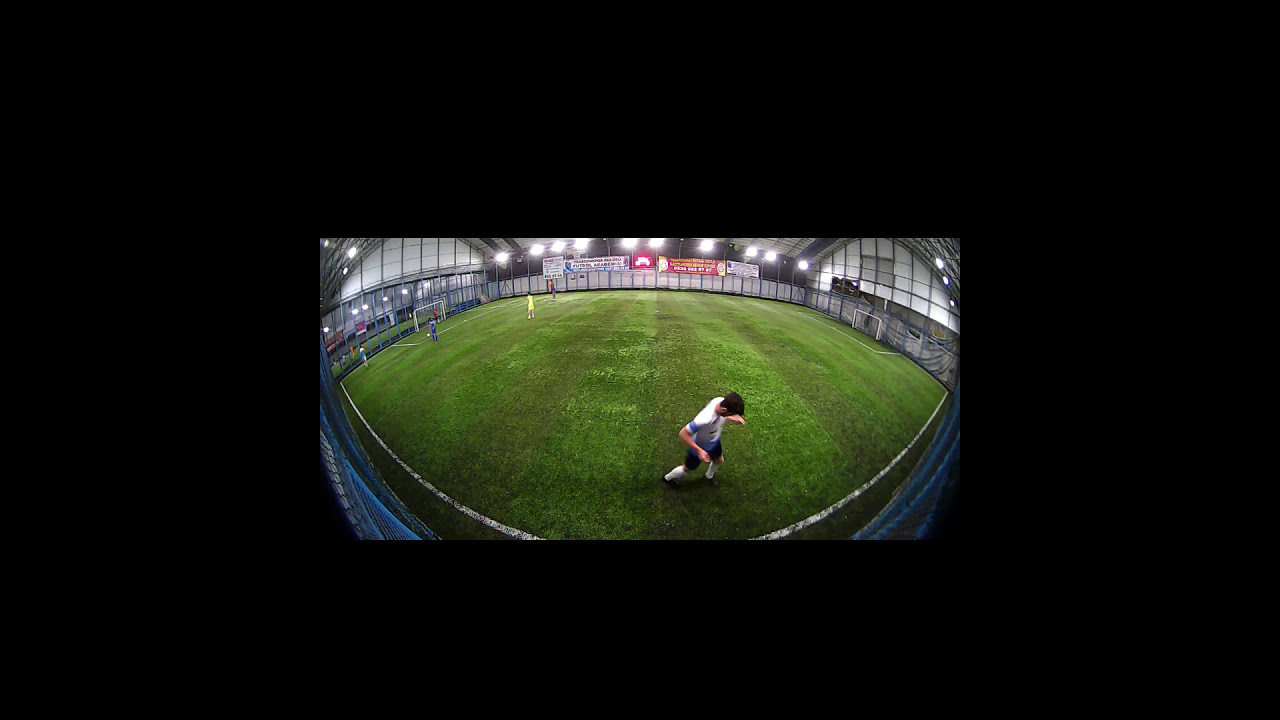This detailed image captures the dynamic scene within an indoor soccer dome. The setting features a long, lush, and impeccably maintained green turf field, dramatically curved due to the fisheye lens or a 360-degree photo effect. Dominating the foreground is a light-skinned individual with dark hair, sporting a white shirt, black shorts, and tall, padded white soccer socks, who appears to be wiping their brow. 

The expansive dome interior is well-lit, with lights affixed to the high ceiling and paneling resembling windows along the sides. To the left, a soccer goal is visible, in front of which four or five people are arranged in a semicircle, several feet apart. Another individual stands inside the goal. 

In the distance, the far end of the dome features numerous advertisements, adding vibrancy to the background. While the fisheye effect skews the entire image, enhancing the curvature of the field, this innovative lens choice makes the additional players and details on the field appear smaller and less distinct.